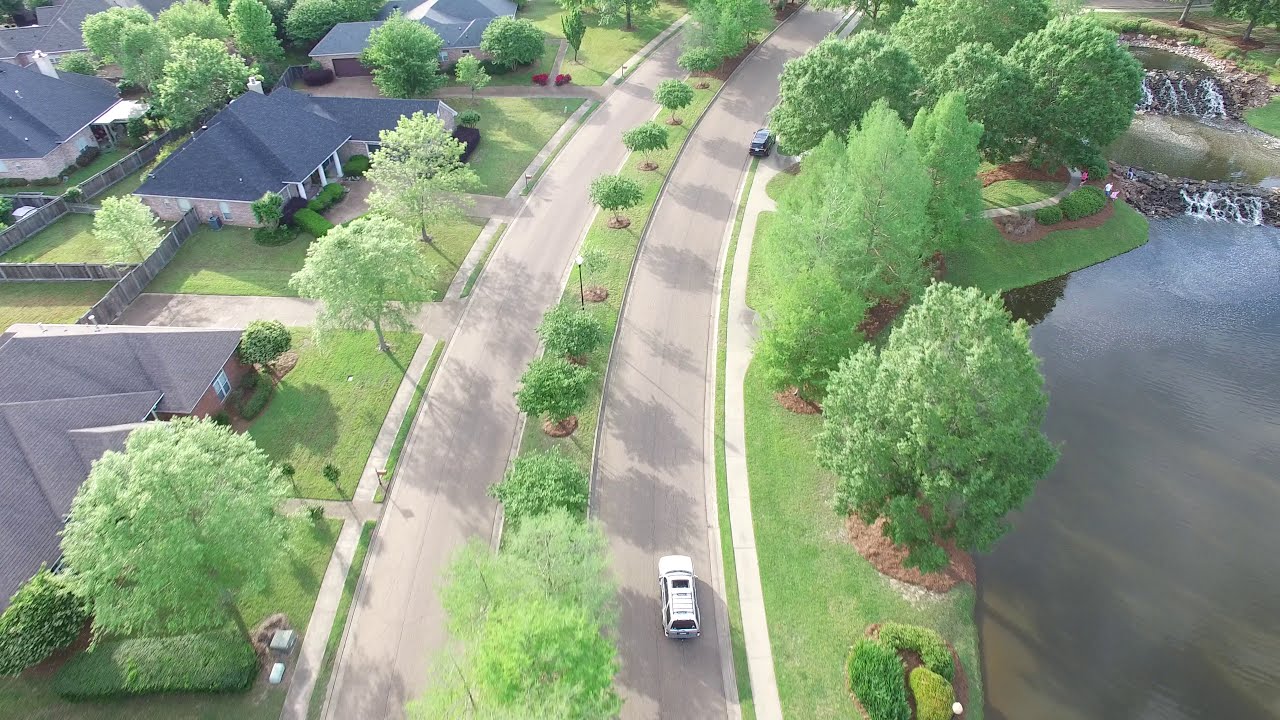This aerial photograph captures a serene residential neighborhood split by a winding road featuring a central divider adorned with small trees. On the left side, there are several sizable single-story and a few two-story houses with distinctive black triangular roofs and brown walls, each with its own manicured lawn and tree-planted front yard. Behind these homes, some backyards are enclosed with fences. On the right side of the road, a white car drives north, while a darker vehicle is parked along the curb. Adjacent to this, a picturesque park area unfolds, featuring a large lake, two small cascading waterfalls situated in the top right corner, and a border of tall trees providing a lush backdrop.